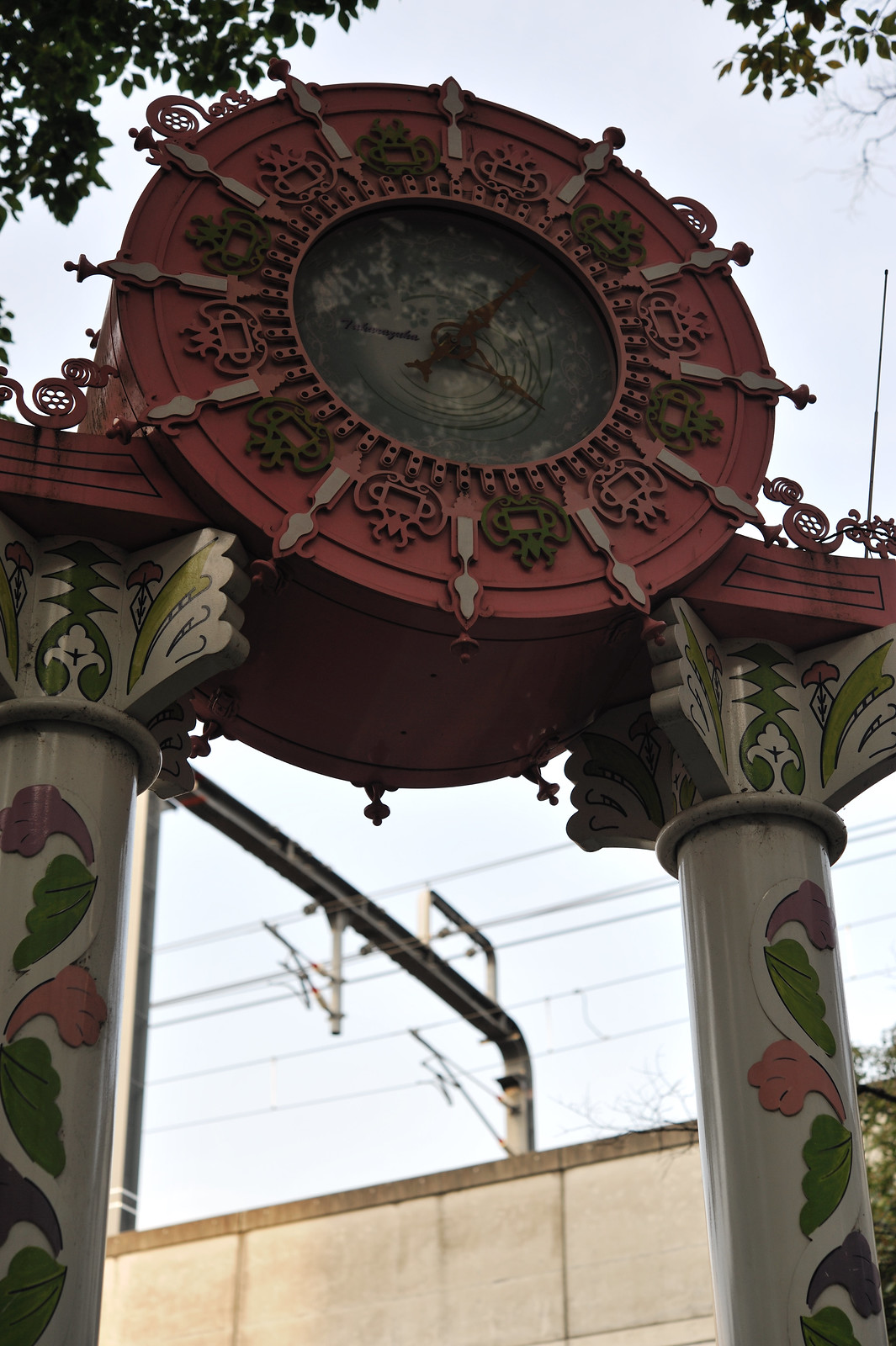The photograph is an outdoor, first-person POV image taken during the day from a tilted upwards angle towards the overcast, light gray sky. At the top of the image, tree branches with green leaves frame the scene. The central focus is a tall, decorative gateway styled in the traditional Chinatown red and green color scheme. Two ornate white columns, adorned with colorful paintings of leaves and flowers, support a large, steampunk-inspired metal clock. The clock, set within a striking red circle, features antique hands and weathered, worn numbers arranged on the outside along with intricate minute notches. Visible behind the gateway are power lines and a concrete wall, adding depth to the composition.